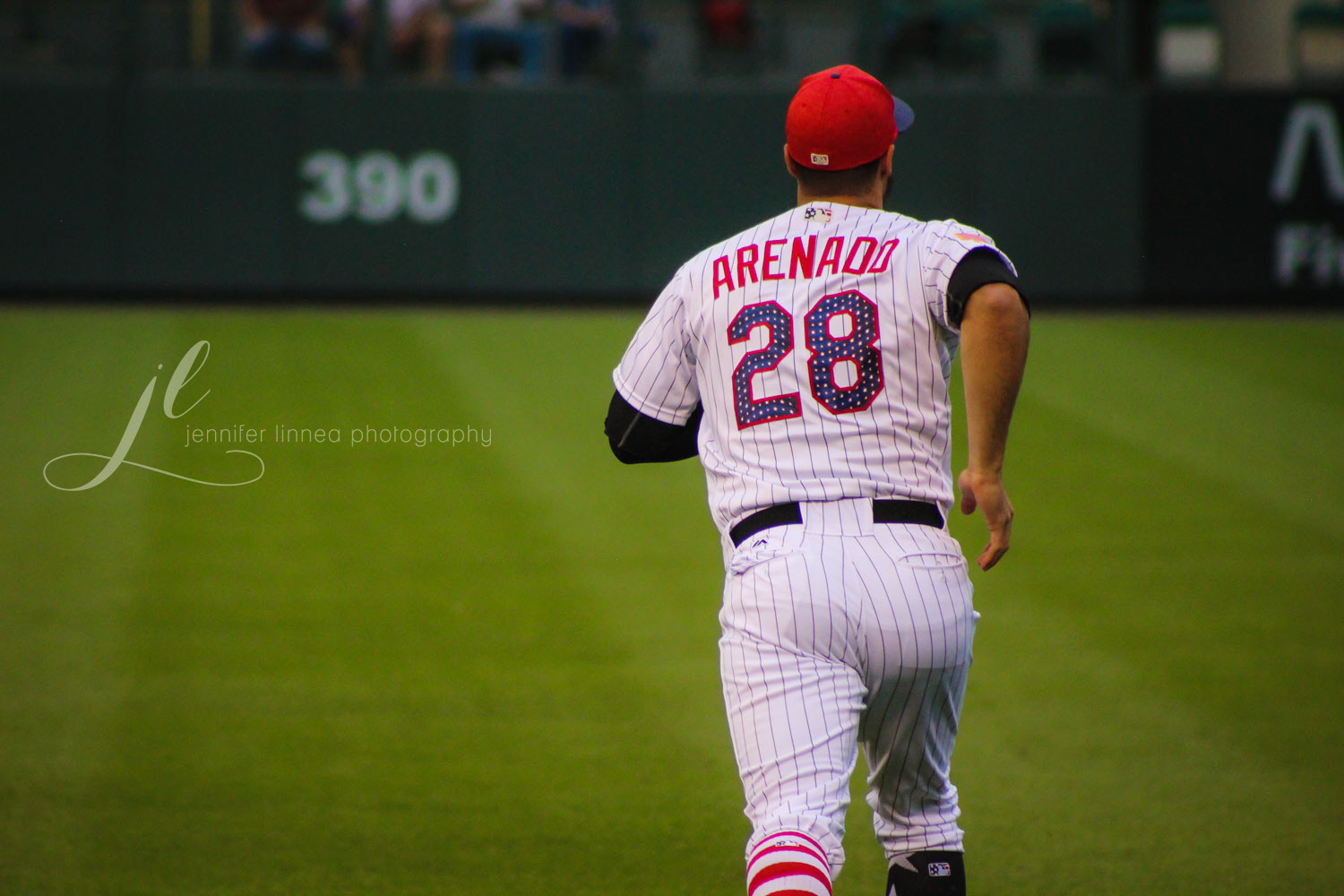The image captures a baseball player, identified by his red and blue hat, running into the field. The hat, adorned with the MLB logo on its back, and his white uniform with thin vertical black stripes emphasize his affiliation. The name "Arenado" is prominently displayed in red letters on his jersey above the number 28. His socks feature a motif of the United States flag, adding a touch of patriotic flair. The background, slightly unfocused and blurred, reveals a dark green wall with the number 390 marked in white. On the left side of the image, the credit "Jennifer Linnea Photography" is visible. The player traverses the meticulously short grass typical of a baseball field, moving away from the camera.